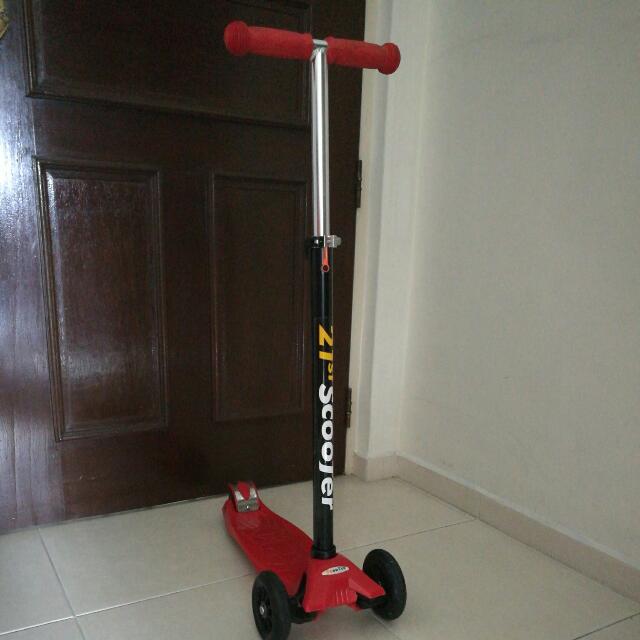This detailed photograph captures an indoor setting, showcasing a three-wheeled scooter prominently placed on white tiles. A dark brown, paneled wooden door serves as the backdrop, providing a stark contrast to the bright colors of the scooter. The scooter features a red base deck attached to two large black wheels at the front and a smaller red wheel at the back, which includes a silver foot-operated brake knob. A sleek black rod rises from the base, inscribed with the text "21st Scooter." Emerging from the center of this black rod is a silver adjustable rod, secured with a clasp. The silver rod culminates in a T-shaped handlebar padded with red rubber grips, enhancing the scooter's vibrant design. This careful arrangement of elements and colors, set against the simplicity of a white-tiled floor and white walls, suggests the photograph was taken in an interior space, possibly an entryway or a similarly minimalist room, prepared for imminent use.